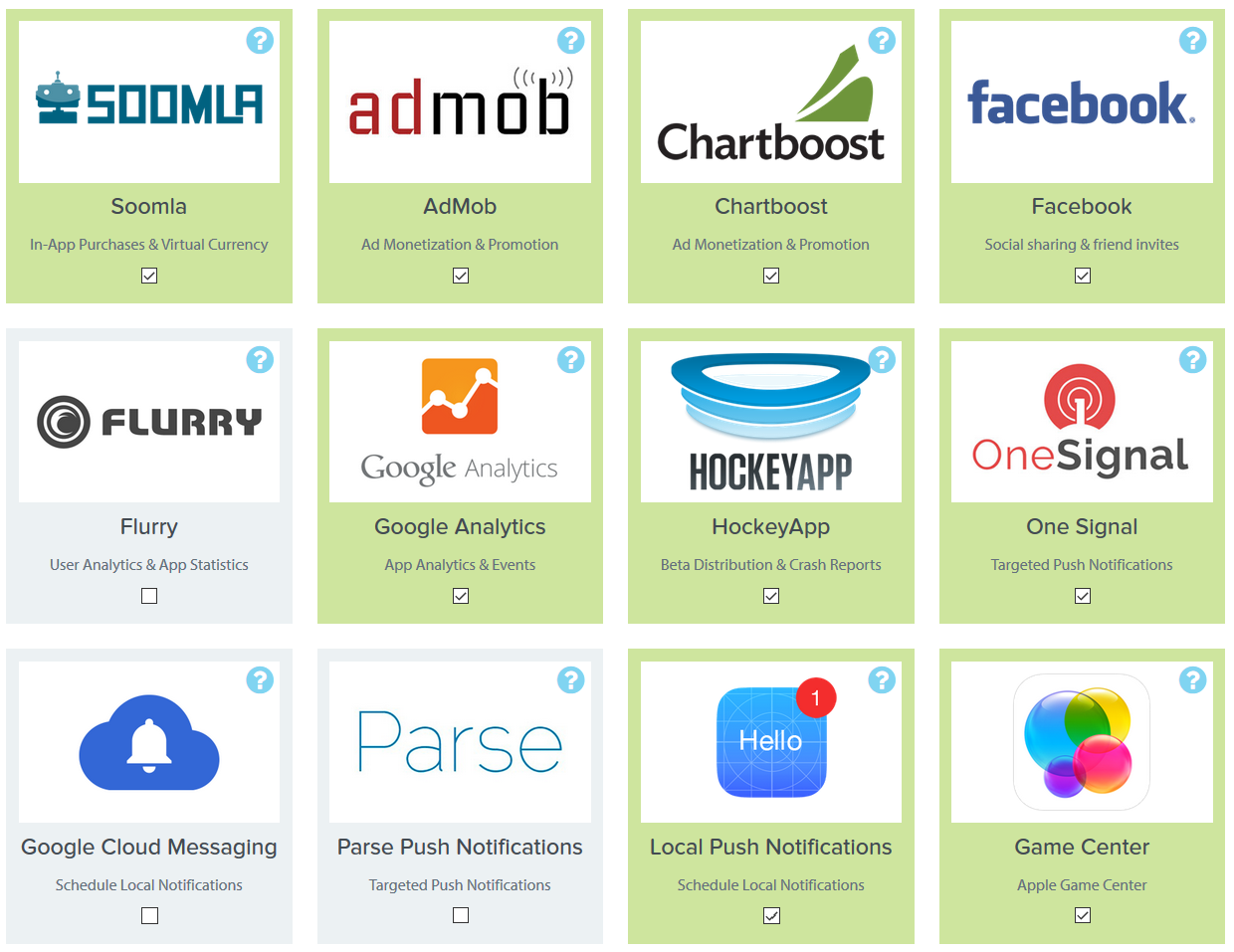This image is a composite screenshot of a webpage displaying a grid of 12 product listings, arranged neatly in three rows of four squares each. Each square serves as a product thumbnail, showcasing the product name and logo in a consistent design format.

- **Top Row (left to right):**
  1. **Sunla:** Encased in a white text box with a green outer box.
  2. **AdMob:** Similar design with a white text box inside a green background.
  3. **ChartBoost:** Follows the same pattern with a green background and a white text box.
  4. **Facebook:** Again, a green background with a white text box.

- **Second Row (left to right):**
  1. **Flurry:** This one deviates slightly, featuring a gray outer box with a white text box.
  2. **Google Analytics:** Returns to the green background with a white text box.
  3. **HockeyApp:** Continues the green and white color scheme.
  4. **OneSignal:** Also follows the green background and white text box design.

- **Third Row (left to right):**
  1. **Google Cloud Messaging:** Another gray background with a white text box.
  2. **Parse:** Reverts to the green background with a white text box.
  3. **Hello:** Maintains the green and white format.
  4. **Game Center:** Concludes the grid with the green background and white text box design.

The entire grid is set against a plain white background, making the green and gray boxes stand out prominently. Each product listing is uniformly styled, featuring the respective logo and name of the product. The overall design is clean and minimalistic, emphasizing the distinct identity of each product through a consistent visual language.